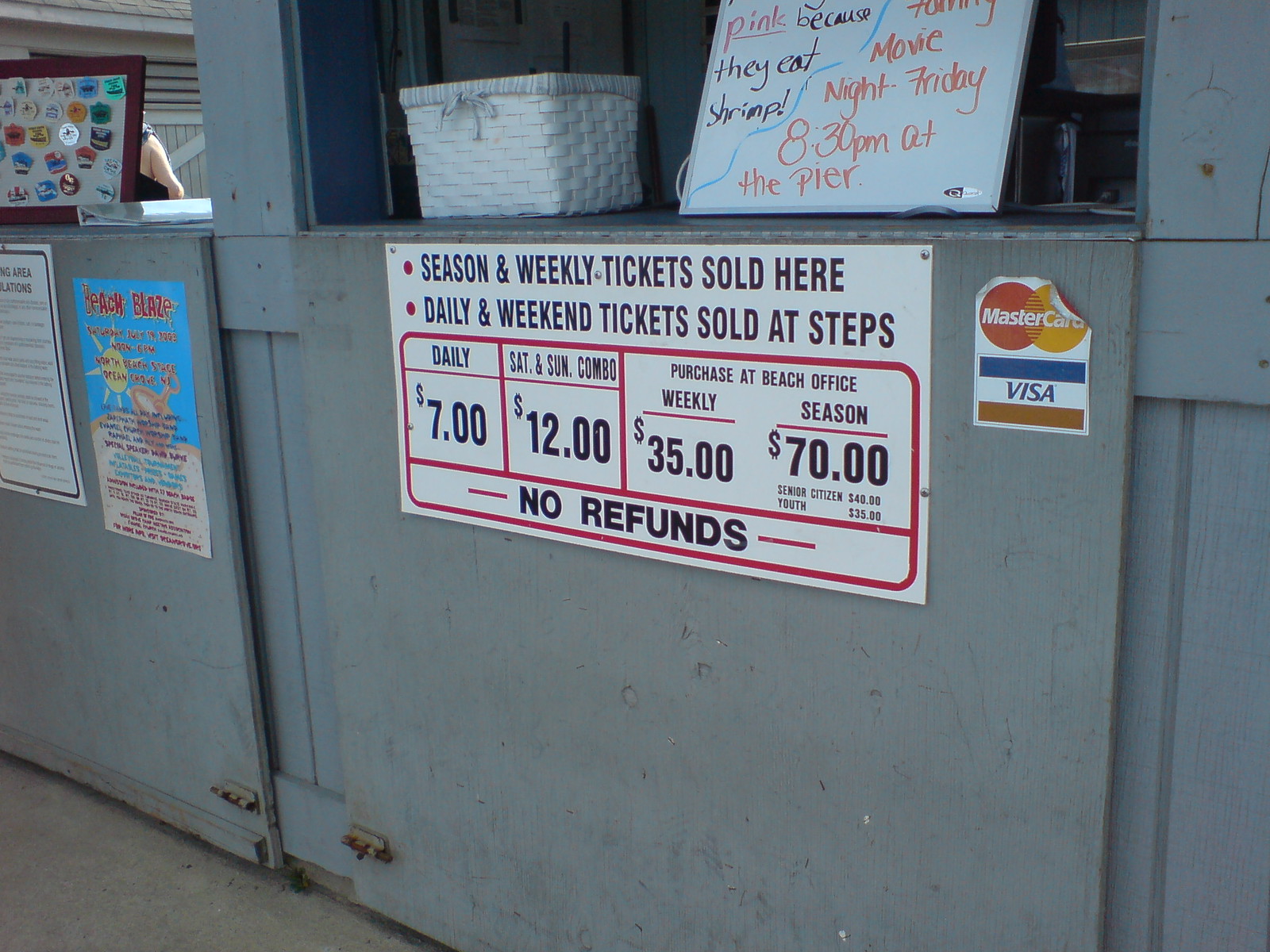The image is an outdoor photograph taken during the daytime, featuring a row of vendor booths on the outside of a store or market area. The booths appear as enclosed, wooden stalls with large panels that drop down to create countertops when open and can be latched and locked up at night. The closest booth has a green, industrial-looking wall with a small opening at the top, implying it might be used for transactions. The booth displays a variety of signs and information. One prominent sign reads, “Pink because you eat shrimp, movie night, Friday, 8:30 p.m. on the pier.” Another white sign with black print details ticket pricing: "Season and weekly tickets sold here. Daily and weekend tickets sold at Steps. Daily tickets are $7. The Saturday and Sunday combo is $12, which can be purchased at the Beach Office. Weekly tickets are $35, season tickets $70, senior citizen tickets $40, and youth tickets $35. No refunds.” Below these signs is a MasterCard and Visa sticker. 

To the left, another booth displays a sign with “Beach Blaze” and event details: "Saturday, July 19, 2003, Noon to 6, North Beach Space, Ocean Grove, New Jersey.” This booth also has a display board with various pins. Adjacent to this display is another sign with regulations, though the precise text is unreadable. The overall scene captures a bustling marketplace environment, ready for commerce and community events.